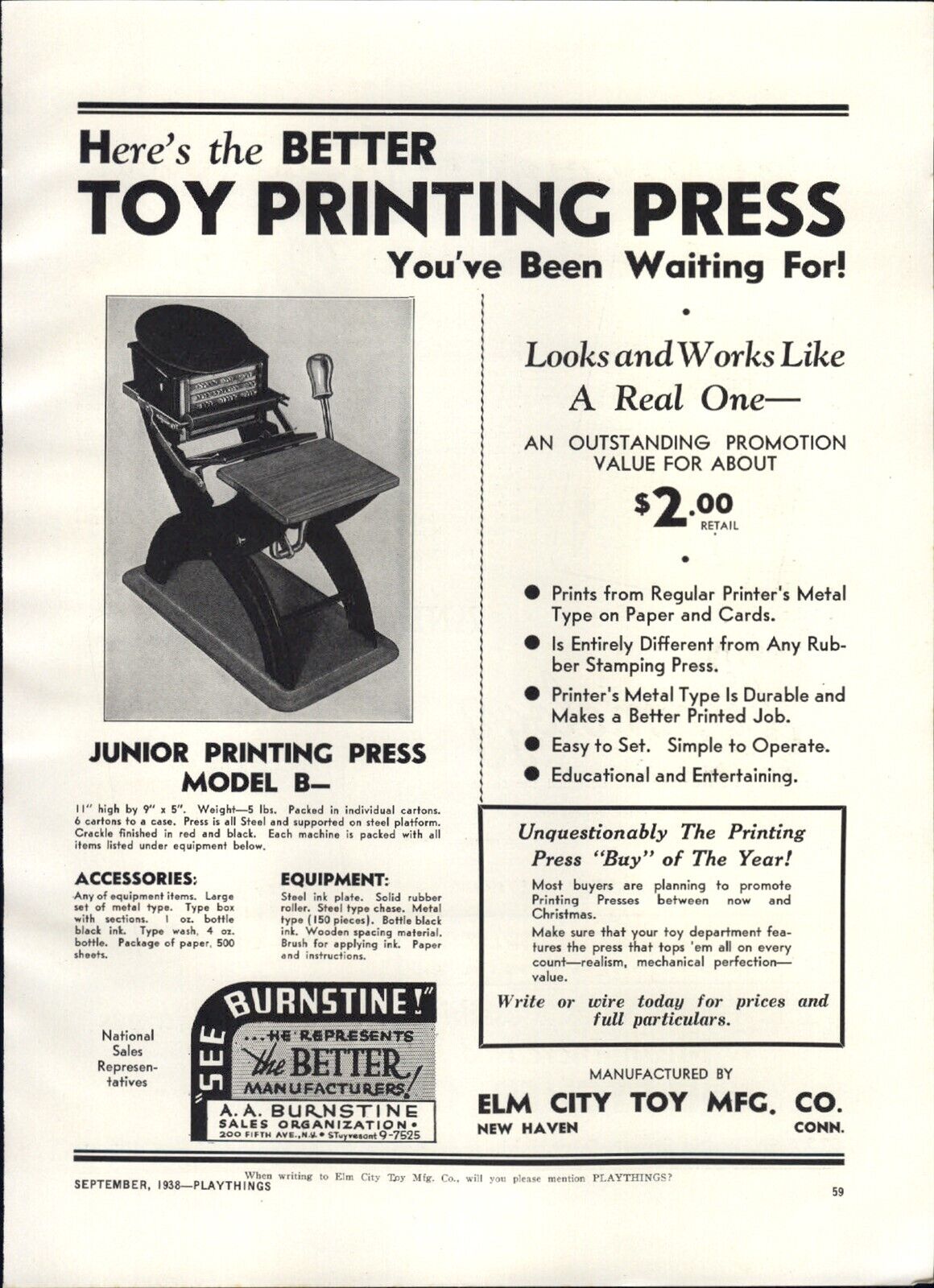Here's a detailed descriptive caption merging all the provided details:

"This black-and-white advertisement from September 1938, featured in Playthings magazine, showcases the 'Junior Printing Press Model B' by Elm City Toy Manufacturing Company of New Haven, Connecticut. Touted as 'the better toy printing press you've been waiting for,' this model notably 'looks and works like a real one' and offers 'an outstanding promotion value for about $2 retail.' The ad emphasizes its function to 'print from regular printers' metal type on paper and cards,' distinguishing it from any rubber stamp machine. The printed job is touted as durable and of high quality due to the metal type used. The press itself is described as being easy to set up, simple to operate, and both educational and entertaining. Measuring 11 inches high by 9 inches wide by 5 inches deep and weighing 5 pounds, each unit is packed in individual cartons, with six cartons to a case, and is supported by an all-steel platform. The accompanying photo illustrates the sleek, steel design of the printing press. Representing the manufacturer is C. Bernstein from A. A. Bernstein Sales Organization at 250 Fifth Avenue, New York. The ad encourages retailers to feature this exceptional toy press in their stores, highlighting its realism, mechanical perfection, and value, especially leading up to Christmas."